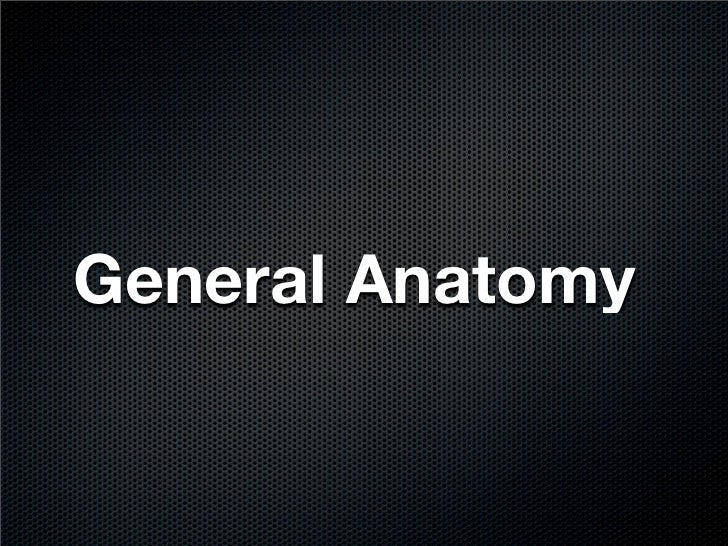The image appears to be a slide from a presentation. It has a predominantly black background with closely packed, tiny silver or black dots, creating a textured effect. In the very center of the slide, large, thick white letters spell out "General Anatomy." The word "General" has a capital "G" with the rest of the letters in lowercase, while "Anatomy" follows the same structure with an uppercase "A." The white text is prominent and includes a subtle black shadow or outline to enhance its visibility against the background. This slide has no other content, making it a straightforward, clear heading, likely designed for emphasis in the presentation. The font size is estimated to be between 18 to 20 points.